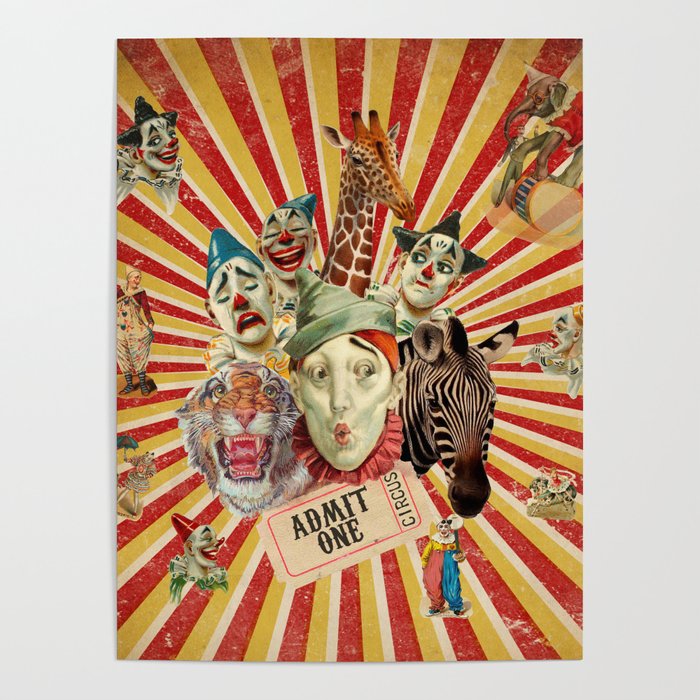The image is a vibrant and detailed vintage-style circus poster. The background is composed of bold red and yellow stripes, accented with white, giving it a lively and dynamic feel. At the center of the poster is a clown with a grayish-green hat and red hair, with a surprised expression on his face. Below him is a ticket stub that reads "Admit One Circus".

Surrounding the central clown are various circus animals and additional clowns. To his left, a tiger roars, showcasing its teeth, while to his right, a black and white zebra stands. Above the central clown is a tall giraffe, adding height and whimsy to the composition.

Scattered around the poster are three more clowns, each displaying distinct emotions: one appears smug, another sad, and a third joyful. Additional clowns don various hats—green, blue cone hats, and even triple black cone hats. Also present is an elephant, balancing on a large drum.

The overall composition of the poster, with its mix of playful clowns and majestic circus animals against a striking striped backdrop, evokes a nostalgic feeling of an old-fashioned circus advertisement.